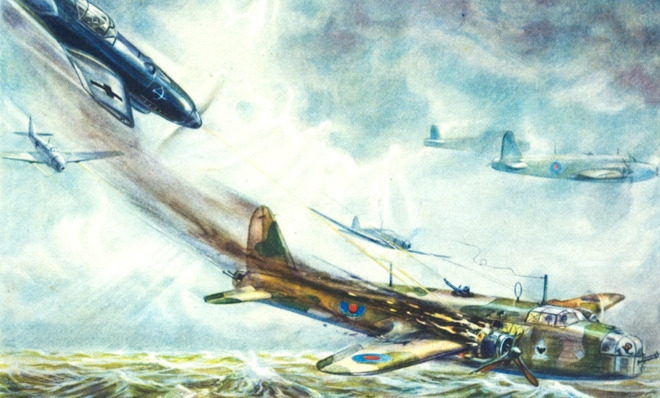This detailed watercolor painting depicts a dynamic wartime aerial battle. At the center, a Japanese fighter plane, identified by the emblem on its wings, is engulfed in flames and descending toward the ocean, leaving a trail of smoke behind it. In stark contrast against the bright central sky, the top right corner of the painting is darker, amplifying the tension of the scene. Surrounding the flaming aircraft are five other planes in varying states of engagement. Some are obscured by clouds, while others are vividly detailed, showcasing their national insignias, such as a British crest on one wing. Two of the planes exhibit aggressive postures, seemingly on the offensive, with one even emitting yellow flashes, indicative of gunfire. Altogether, the painting captures the chaos and intensity of an aerial dogfight, with bombers and fighter planes set against a backdrop of clouds and the bright sun, all intricately rendered with green and yellowish-green patterns on some aircraft, adding to the historical ambiance of the scene.